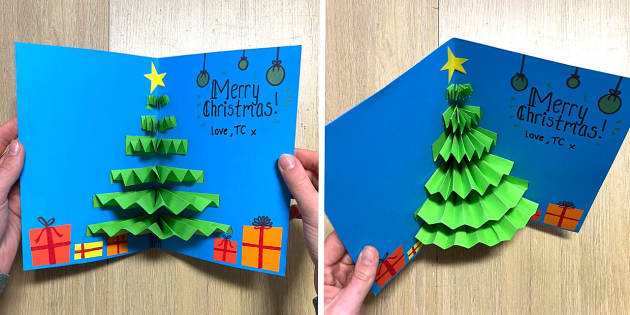In the image, there are two side-by-side photos of a handmade Christmas card crafted from blue construction paper, showcased on a light brown wooden table. The card is open, revealing a pop-up Christmas tree in an accordion design made from green construction paper. A yellow star adorns the top of the tree, while illustrated paper presents, including variously colored boxes—orange, red, yellow—occupy the bottom of the card. In the upper right corner, the card is inscribed with "Merry Christmas, Love TC." Snowflake decorations and three hanging gold ornaments add festive flair. In the photo on the left, a person's thumb and forefinger are visible, holding the card flat, fully displaying the 3D tree. In the photo on the right, the card is angled upright towards the bottom right, supported by a hand visible in the bottom left corner. The detailed presentation captures the intricacy and personal touch of the holiday greeting.